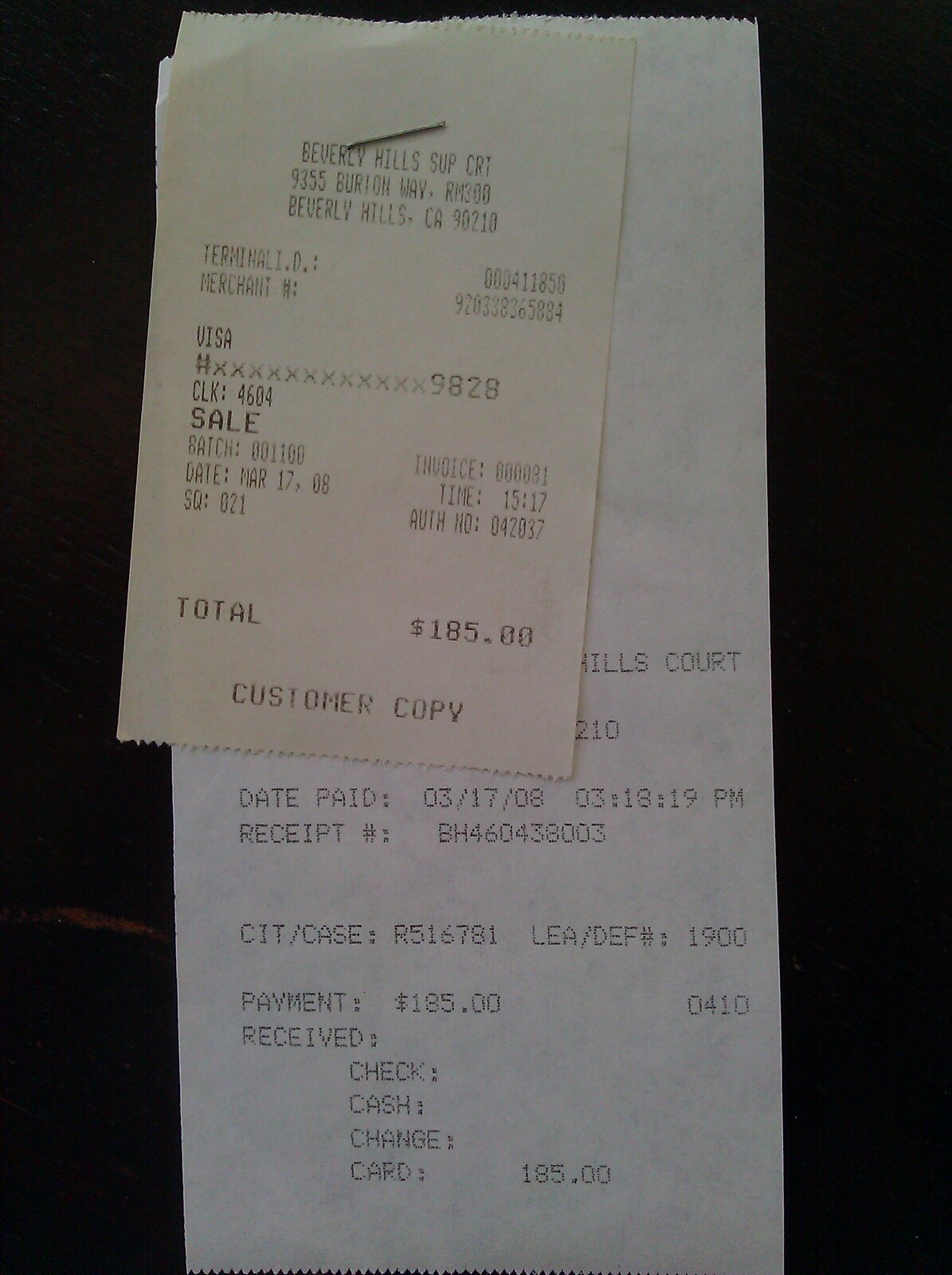On a stark black background, a detailed image showcases a white receipt with black print, prominently featuring the header "Beverly Hills Superior Court." The document itemizes a Visa charge amounting to $185, labeled as "Customer Copy." Displayed above, a second receipt, also indicating the same charge, is visibly stapled to the first one. The transaction details are meticulously printed, noting the payment date as March 17, 2008, at 3:18:19 p.m., alongside a specific receipt number. Both receipts underline the identical amount of $185 paid by card, cementing the thorough nature of the documentation.